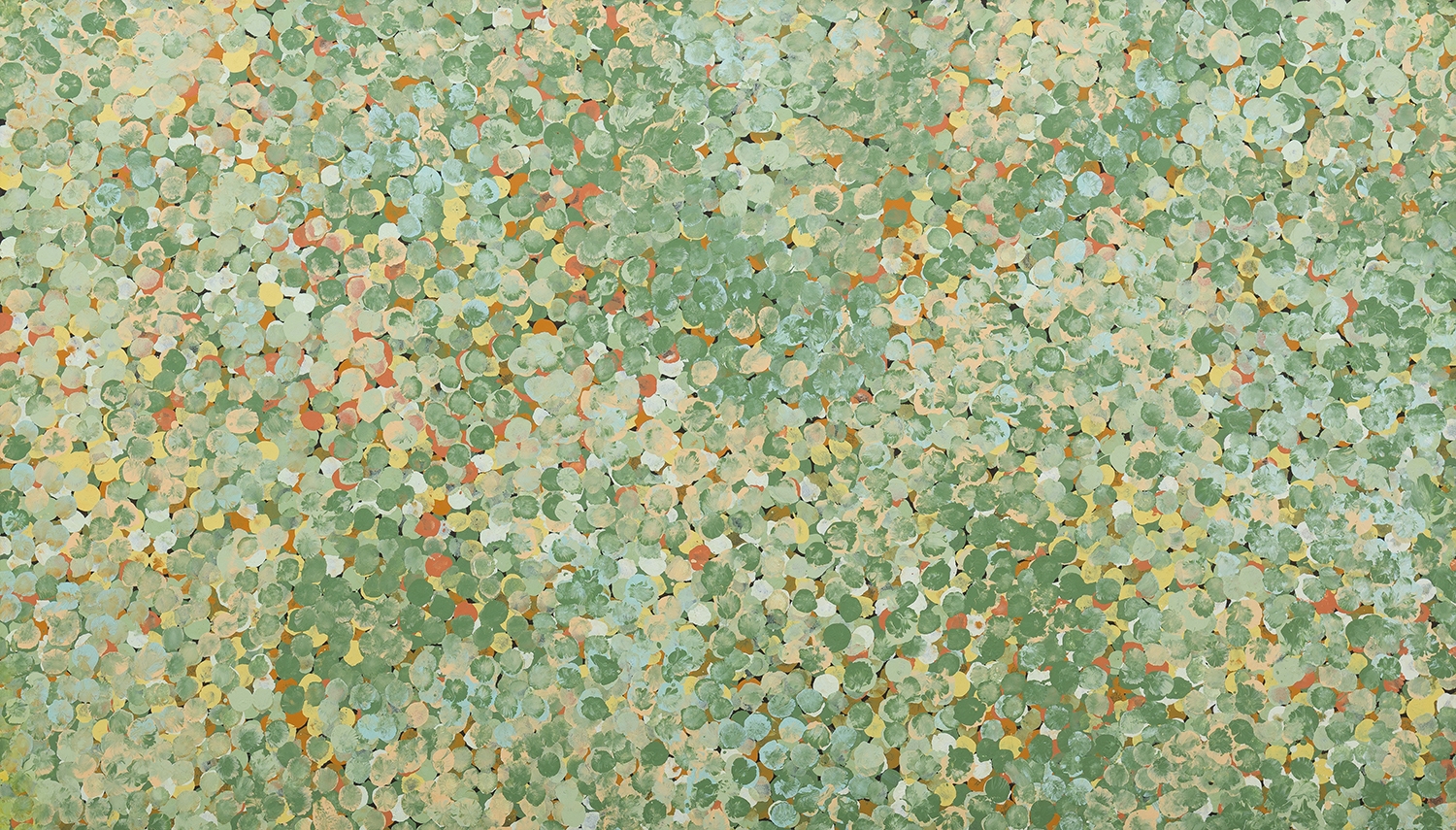The image depicts a detailed and richly textured artwork or photograph, showcasing an intricate composition of small, circular shapes resembling beads or petals. These circles vary in color ranging from light green, medium green, to muted yellow hues, with occasional rust-colored and whitish-gray accents. The circles appear to be meticulously layered, creating a sense of depth and movement across the entire surface. Although they seem to be punched out like confetti, the careful arrangement suggests an artistic intention, mimicking a natural scatter of elements most akin to flower petals or glass beads reflecting light. The background is predominantly concealed underneath the multitude of circles, with yellow hints suggesting an underlying yellow surface. This visually captivating piece covers the entire field without forming any discernible pattern, person, place, or thing, making it an abstract and engaging focal point for minimalist decor.